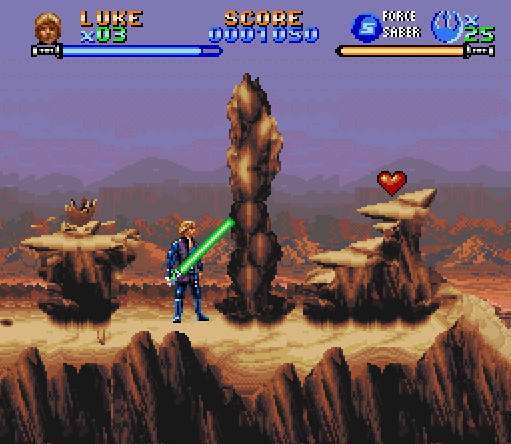The image showcases a video game screen where a warrior-like character, identified as Luke, stands on rugged, mountainous terrain. Luke wields a green lightsaber in his right hand, suggesting a connection to the 'Force Saber' as indicated in the game's interface. In the top right corner, the text "Luke x03" signifies his current lives or attempts remaining. Below, his score is displayed as 0001050. Additionally, Luke's power meter stands at "x25." A heart icon, likely representing health or an extra life, rests on one of the rocky ledges in the background, ready to be collected. The overall scene captures an intense moment in the gameplay, emphasizing the character's readiness for battle and the strategic elements involved.